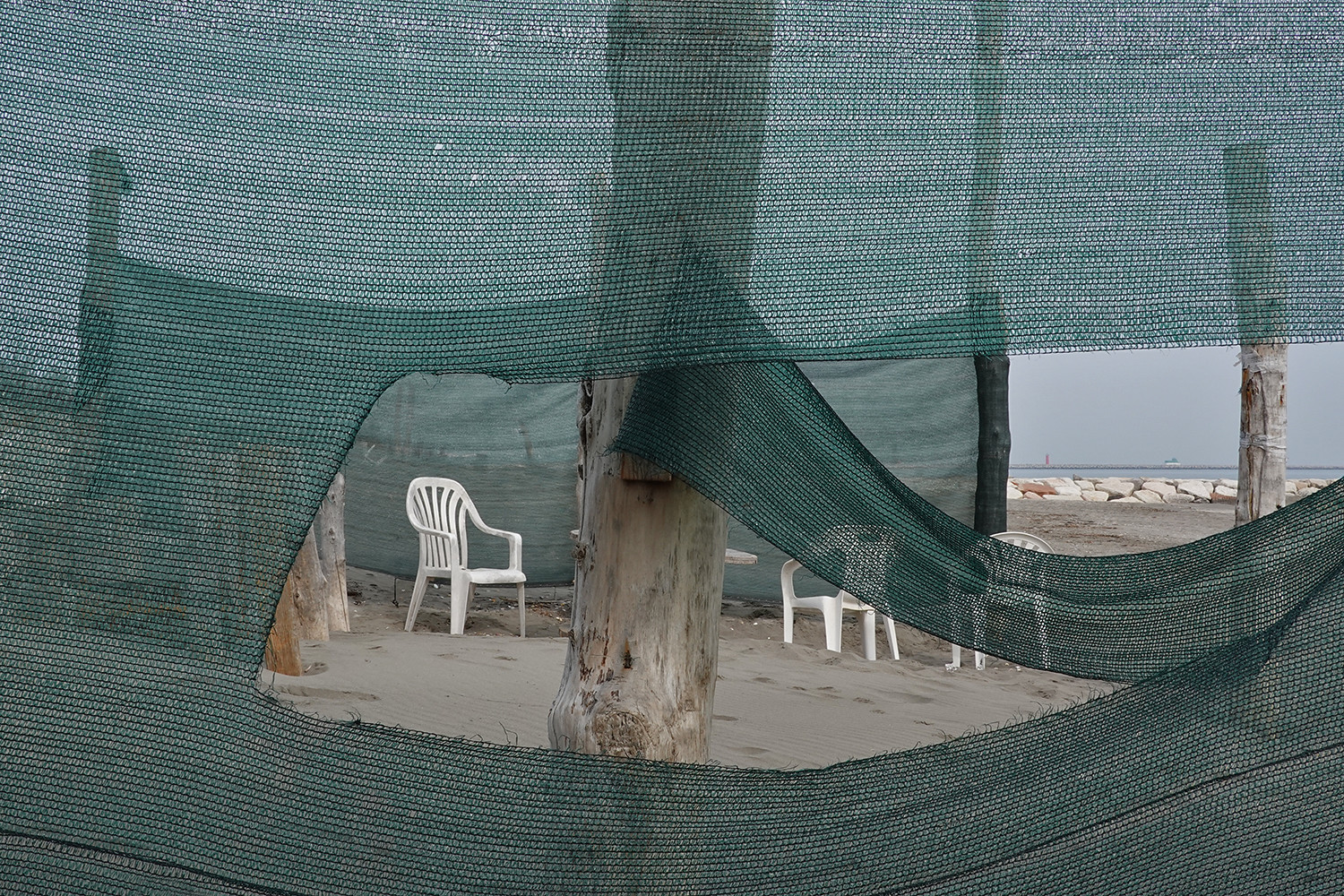The photograph captures an outdoor seating area adjacent to a beach on an overcast day with a solid light gray sky. In the foreground, there are multiple wooden posts, retaining some natural textures like knots, that are embedded into the hard-packed sandy ground, creating a framework for a green canvas-like fabric privacy wall. This material forms a sort of makeshift tent or enclosing, with an opening visible between a pair of posts. Inside this area, three white plastic lawn chairs encircle the edges of a partly visible table, which is partially obscured by one of the wooden posts. The left side of the scene is complemented by a smaller arrangement of logs forming a modest barrier. 

Beyond this enclosed space, the scene features extensive brown sands with a large expanse of water in the distance, possibly a wide river or sea, marked by white flat rocks forming a ledge or jetty that extends into the water. The outlines of tall grass, akin to those on sand dunes, are faintly visible through the green fabric on the left side of the image. Far across the water, there is a suggestion of a red lighthouse and a possible ship, adding more depth to the distant horizon.